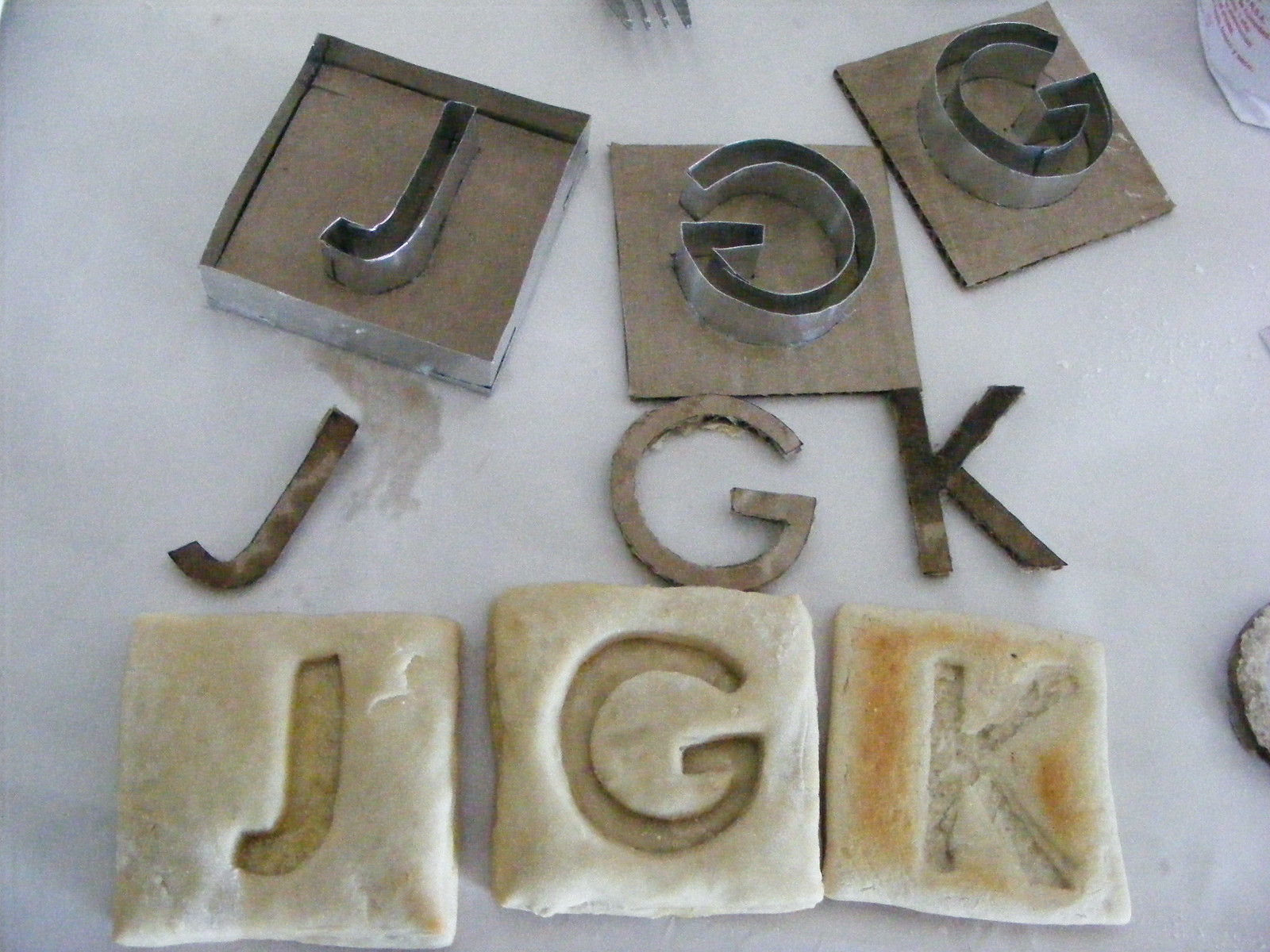The image displays an arrangement of cookies or biscuits and stenciled letters against what appears to be a white table. At the bottom, there are three square-shaped cookies or biscuits, each with a letter imprinted using stencils: 'J' on the left, 'G' in the center, and 'K' on the right. Above these cookies, you can see the stenciled letters that were likely used to create the impressions. At the top, neatly lined up, are the cookie cutter stencils, each matched with the letters that were removed and arranged just below them. Additionally, there is a letter J in an open square box, an inverted letter G on a brown square base, and the correct G on another brown square base. The background includes a partially visible white bag with red lettering, possibly flour, located at the top right, and a fork tip peeking in at the very top of the frame. To the bottom right, there's another indistinct object that could potentially be another cookie. The meticulous arrangement and the letters provide an interesting, layered composition focusing on both the baking process and the final product.